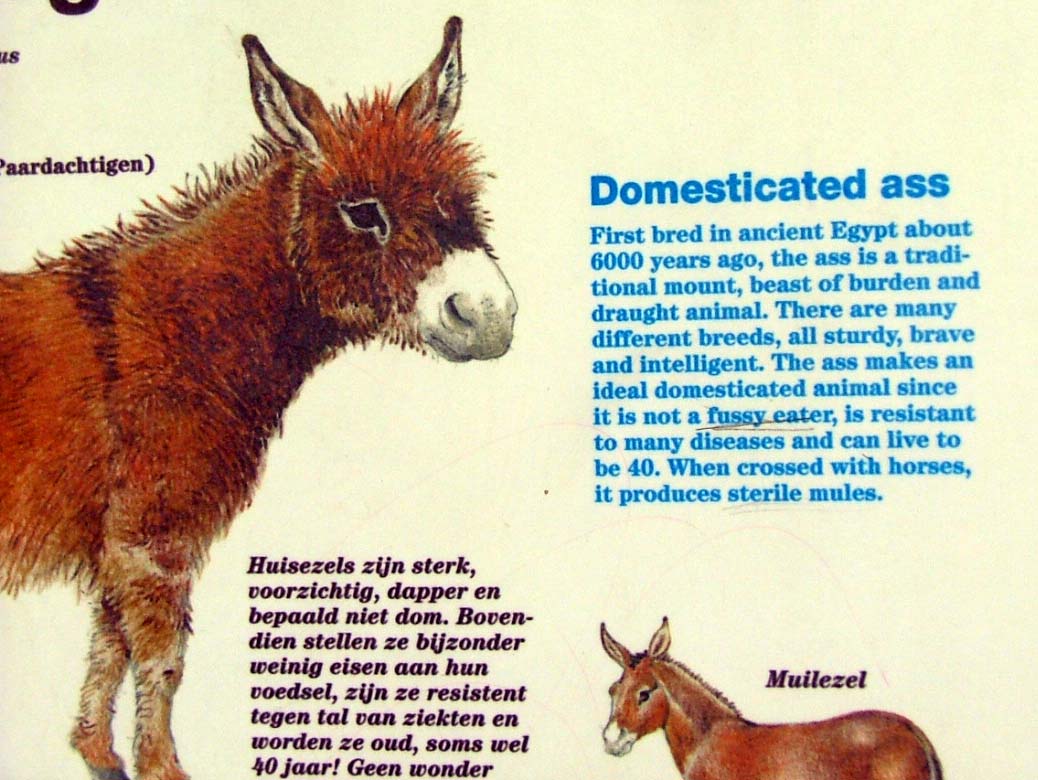This detailed, informative poster depicts donkeys through a blend of drawings and textual descriptions. The main image centers on a brown donkey with a white nose and inner ears, black eyes with white rings, and dark brown legs transitioning to white at the bottom. Its head faces right, prominently displaying its sturdy, upright ears. The background is white, and to the side of the donkey, there is German text providing additional details.

A large blue heading reads, "The Domesticated Ass," followed by a comprehensive paragraph in English. This text explains that the domesticated ass, commonly known as the jackass, was first bred in ancient Egypt around 6,000 years ago. These animals have been utilized traditionally as mounts, beasts of burden, and drought animals due to their sturdy, brave, and intelligent natures. They are resilient to many diseases, not picky eaters, and can live up to 40 years. Additionally, crossing them with horses produces sterile mules.

Below this paragraph, a partial depiction of a mule appears, with its light brown body and white nose. Its head faces left while its tail points to the right, and its ears are erect and pink. Above this depiction, the word "MUILEZEL" is inscribed, highlighting the visual transition from donkey to mule. The poster combines striking visuals with thorough, albeit multilingual, information to educate viewers about these remarkable animals.